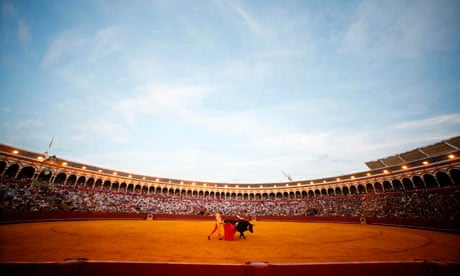The photograph captures a contemporary and densely packed outdoor stadium during a Spanish bullfight. The panoramic view shows a large, round, open-air arena with endless rows of indistinguishable spectators filling the stands. Above this bustling scene, the sky takes up more than half of the top half of the picture and is a pure blue adorned with wispy white clouds. You can see the curving edges of the coliseum-like structure, which features numerous arches, likely made of stone or wood, and lit by orange lights.

In the center of the field, covered in reddish-brown dirt, stands a matador clad in a vibrant yellow suit with a red flag. The matador is depicted engaging a dark black bull, which has already been pierced by several spears. The bull is captured mid-movement, with its legs upright, appearing to slowly advance past the matador. The overall hues of the arena, field, and the matador’s costume blend seamlessly into a spectacle of intense colors and textures, reflecting the drama and tradition of the bullfight.